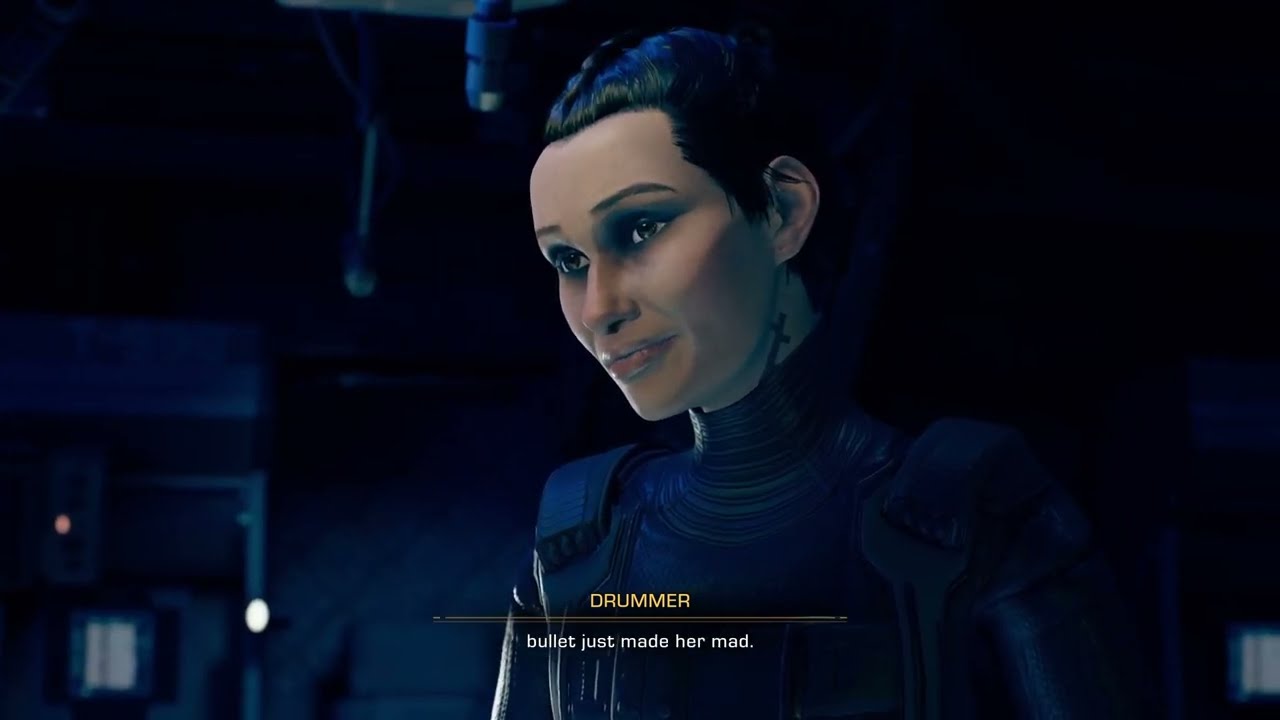This is a horizontal rectangular image that appears to be a screenshot from an animated video game. The scene is set inside a dark building, with a background that fades to black and dark blue tones, making it difficult to discern specific details beyond the central figure. The figure is an animated female with slick, short black hair and brown eyes adorned with blue eye shadow. She has a cross tattoo on the side of her neck. The woman's body is positioned to face the viewer, but her head is turned to the left. She is dressed in what appears to be a dark gray or dark blue, skin-tight futuristic uniform or armor that extends halfway up her neck. At the bottom-center of the image, yellow text in all caps reads "DRUMMER," with a horizontal yellow line beneath it. Below the line, white text states, "BULLET JUST MADE HER MAD." There is a faintly visible corridor or doorway in the bottom left-hand corner of the image, highlighted by lights on the ceiling, suggesting a futuristic setting.